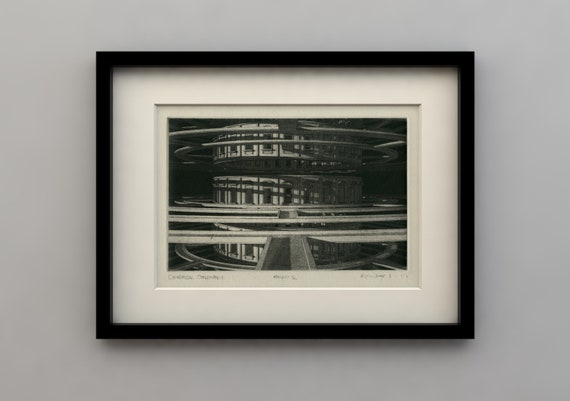The artwork on the light gray wall features a black-framed, matted photograph with a thick white border and a smaller inner border. The image itself, rendered in black and white, depicts a futuristic, multi-level, round building reminiscent of a parking garage or observatory, with several rings or pathways encircling it. The building has three distinguishable levels, each adorned with a continuous row of doorways or windows. Despite some illegible text signed and dated beneath the photo, the overall design is intricate and evokes a sense of depth and complexity.